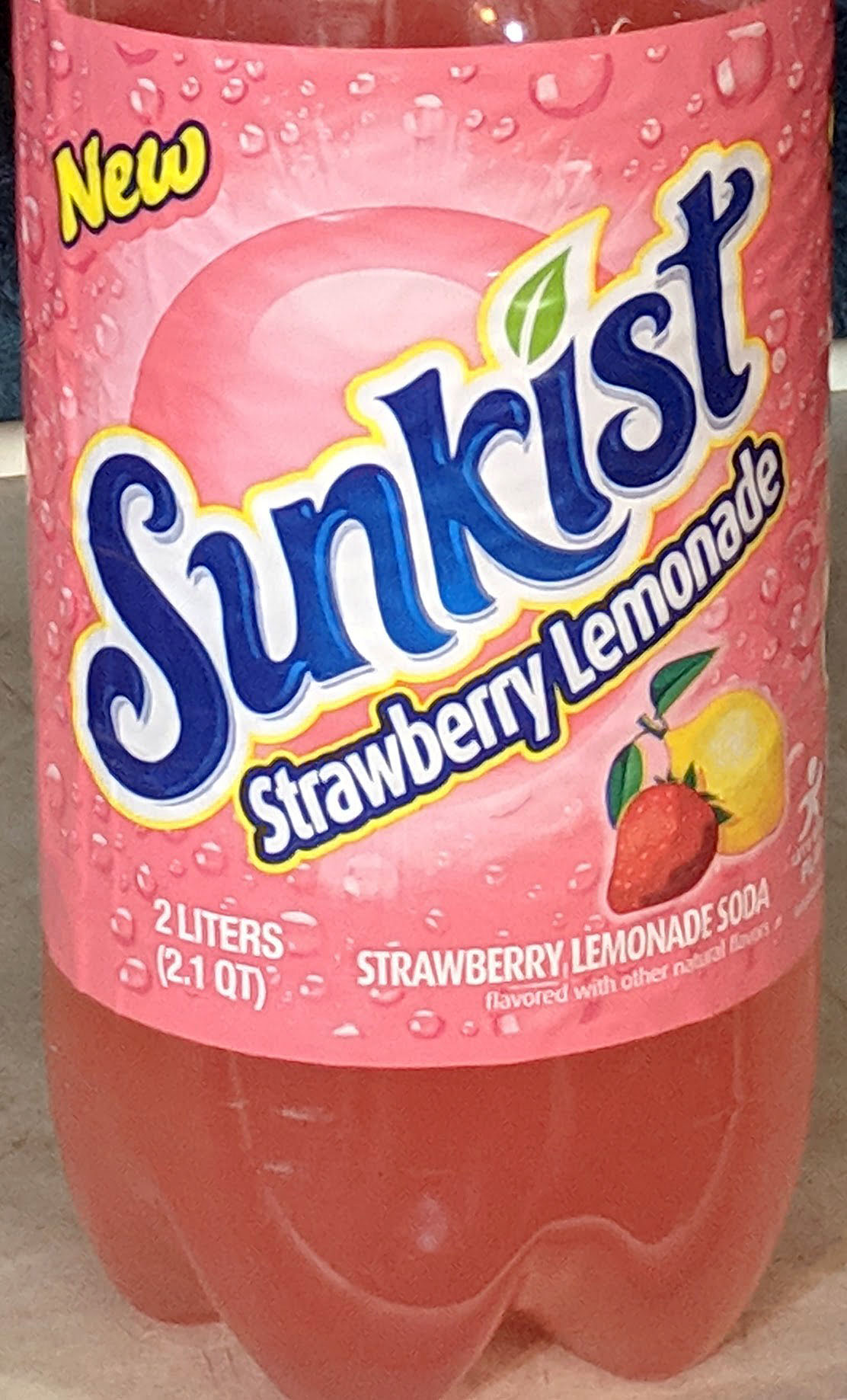A rectangular image showcases a 2-liter bottle of Sunkist Strawberry Lemonade Soda. The prominently featured label, set against a light pink background, displays the Sunkist logo in bold, cursive blue lettering outlined in white and yellow, with a distinctive leaf as the dot over the 'i.' Below the logo, "Strawberry Lemonade" is written in non-cursive blue and yellow-outlined text. The bottom right corner of the label is adorned with vibrant illustrations of a lemon and a strawberry, emphasizing the flavor. Just beneath the name, the label informs that it is "Strawberry Lemonade Soda flavored with other natural flavors." The rich, darker pink hue of the beverage itself is visible below the label. Notably, the upper left corner of the label features the word "New," highlighting the product's recent introduction.